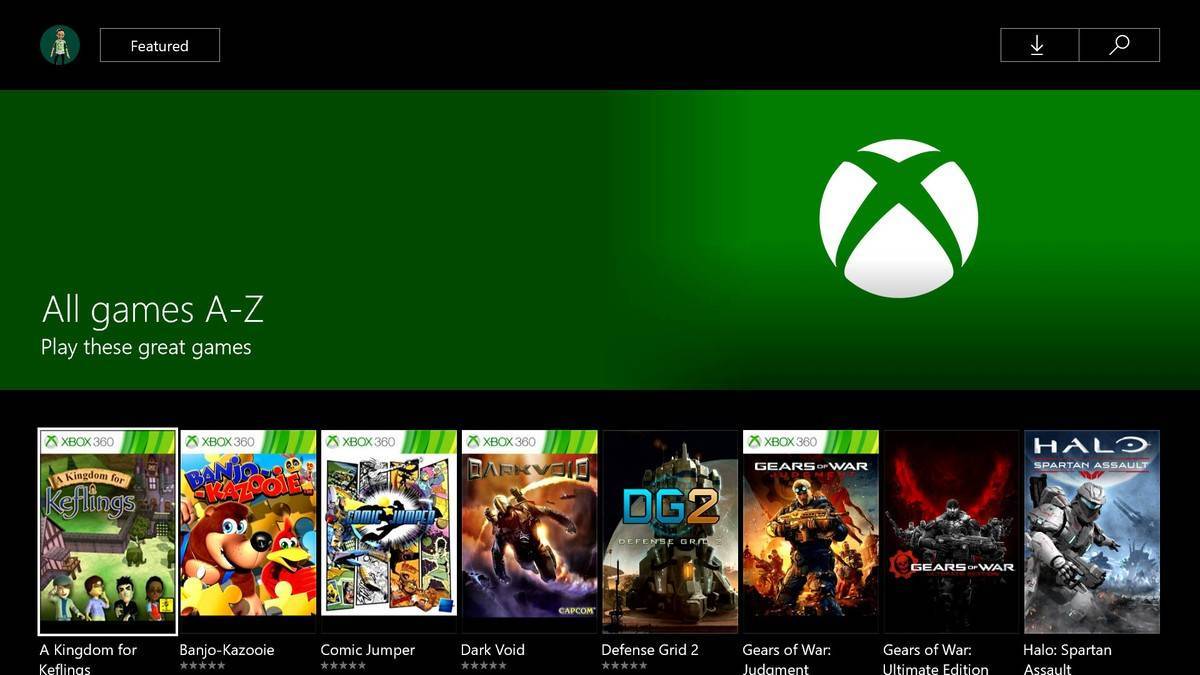The image is a detailed screenshot featuring a predominantly green background that transitions from darker on the left to lighter on the right. At the very top of the screen, there is a wide horizontal rectangle spanning the entire width. In the upper left corner of this rectangle, an icon is displayed. To its immediate right, there's a black button outlined in light gray, labeled "Featured" in white text.

Toward the right side of the rectangle, two additional buttons are visible: one labeled "Download" and another featuring a magnifying glass icon. 

Below this top border, an extensive horizontal green rectangle stretches across the screen. In the lower-left corner of this section, bold white text reads "All Games A-Z," with a secondary line underneath stating "Play these great games" in white. 

On the right of this section, there's a white circle containing a green "X" that extends to the edges of the circle.

Beneath this, a large black rectangle showcases a list of games, each represented by a horizontal rectangle featuring an image of the game. There are a total of eight games displayed in this list, with each game title positioned underneath its respective image. The first, second, third, and fourth games show star ratings below their titles, while the last three games do not have visible star ratings due to the screen being cut off at the bottom.